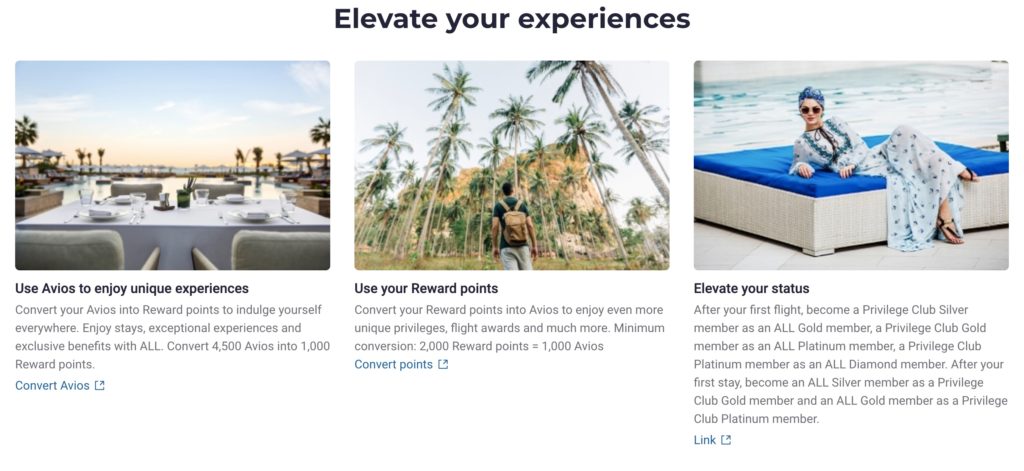This image is part of a triptych advertisement promoting a luxury vacation experience through the use of Avios and reward points. The first image features a stunning sunset with a beautifully set table in an exquisite location surrounded by palm trees. The text alongside reads, "Elevate Your Experiences. Use Avios to enjoy unique experiences. Convert your Avios into reward points to indulge yourself everywhere. Enjoy stays, exceptional experiences, and exclusive benefits. Convert 4,500 Avios into 1,000 reward points." There is a clickable area labeled "Convert Avios" for further action.

The second image showcases a picturesque scene with numerous palm trees, a man carrying a backpack, and a majestic mountain in the background. The accompanying text states, "Use Your Reward Points. Convert your reward points into Avios to enjoy even more unique privileges, flight awards, and much more. Minimum conversion: 2,000 reward points equals 1,000 Avios." This image also includes a blue clickable area titled "Convert Points."

The third image depicts a woman relaxing on a lounge chair beside a serene water body. The text above her notes, "Elevate Your Status," followed by a paragraph detailing the conversion process and benefits of this program. There's a final link for users to convert their points, completing the cohesive and inviting promotional layout.